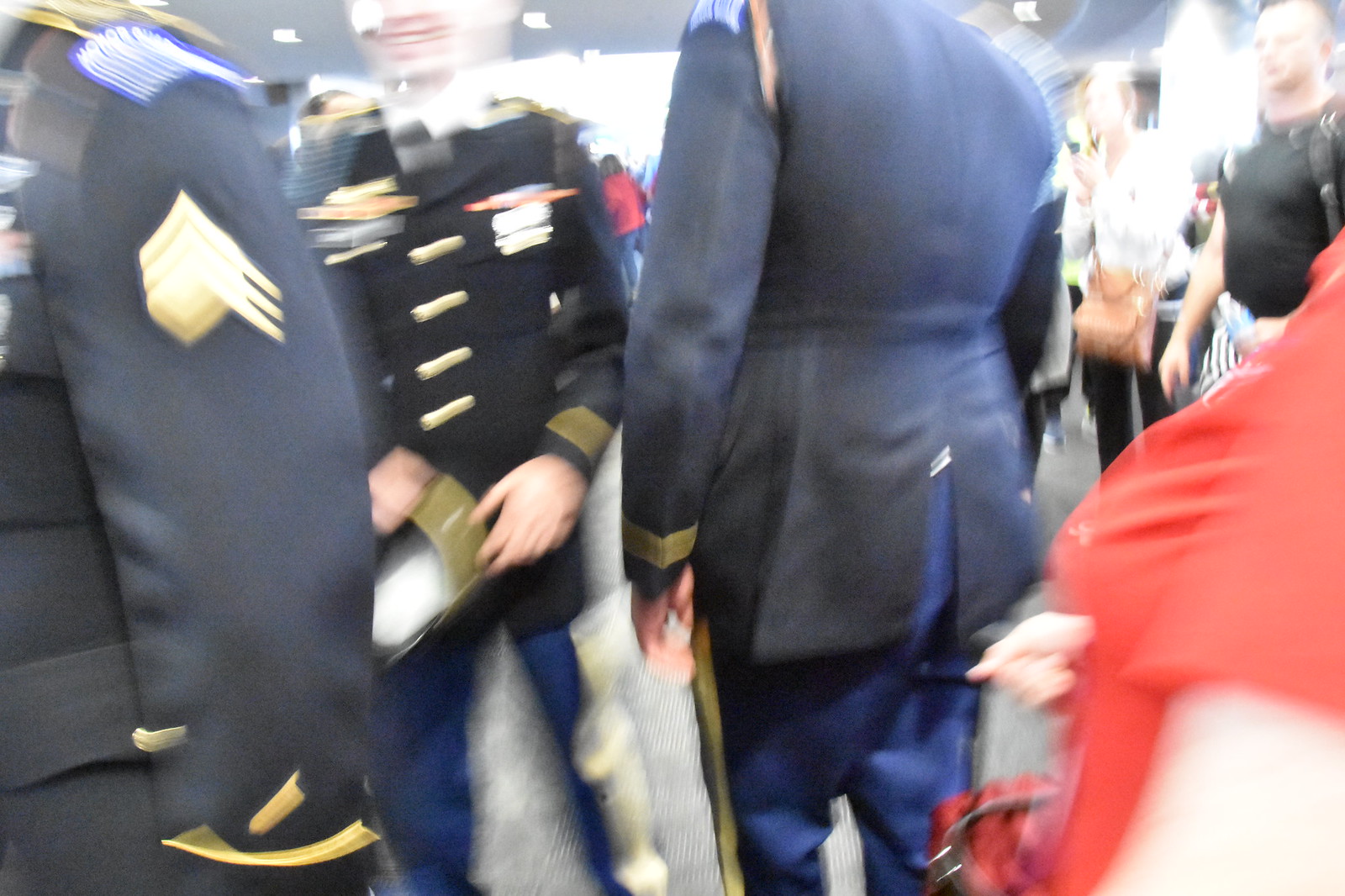In this blurry photograph, a bustling scene appears to revolve around a gathering of military personnel, potentially at a formal event in a large public space like an airport. Dominating the center, the back of an officer clad in a long, dark blue jacket with gold trim around the wrists and a gold stripe down the sides of his matching blue pants catches the eye. This individual, whose uniform also displays a badge on the arm, further features a distinctive slit in the jacket. Flanking him is another officer, visible from the front but obscured from the nose up, donning a similar blue uniform adorned with gold buttons and various pins and awards. He smiles while holding a captain's hat, his attire mirroring the gold-striped blue pants of his counterpart. To the left, the partial arm of yet another officer also reveals the same yellow-striped blue jacket adorned with additional gold and blue patches. The background teems with people, including a woman in a black shirt paired with white and black striped pants and another individual in a red dress. Among the crowd, one can also spot a lady wearing a white shirt and black pants, carrying a large brown purse, adding to the impression of a busy, perhaps ceremonial occasion.